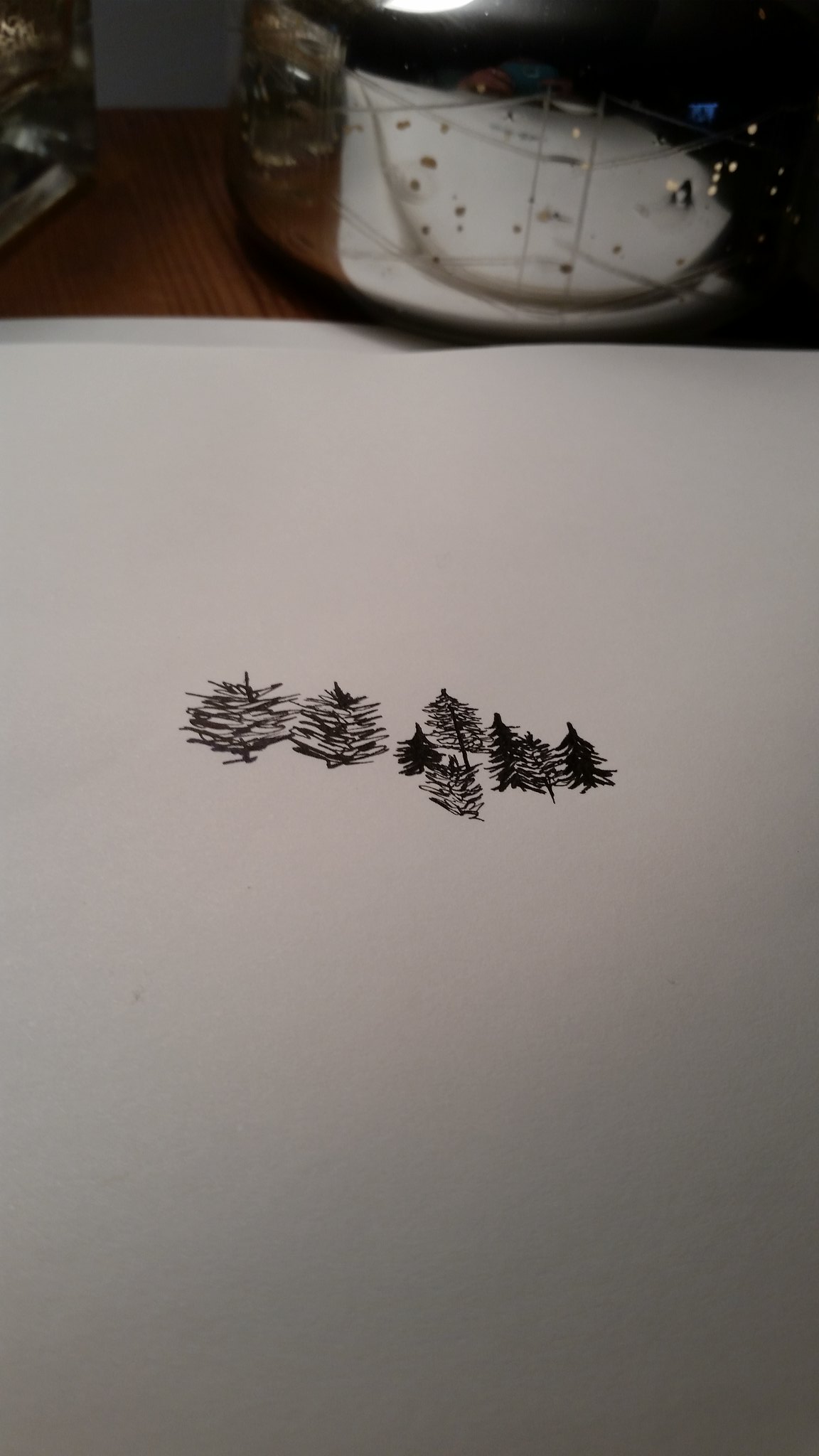The image captures a zoomed-in view of a brown wooden surface, likely a table or counter, adorned with various objects. At the center of the frame lies a white piece of paper with seven small tree drawings in black ink. These trees vary in thickness and darkness; some are pine trees with very dark shading on the right, while those on the left are broader. A shadow on the paper suggests the use of a camera flash. To the right of the frame, a reflective metal object displays the reflection of hands with gold rings and a turquoise-colored camera. Above the paper, there is a white object, possibly a clutch or pocketbook, with gold specks on it. Behind this, partially visible at the top, is another object featuring brown circles and silver lines or strings. The reflective light towards the upper part of the image adds a shimmering effect, potentially from a glossy or metallic surface.